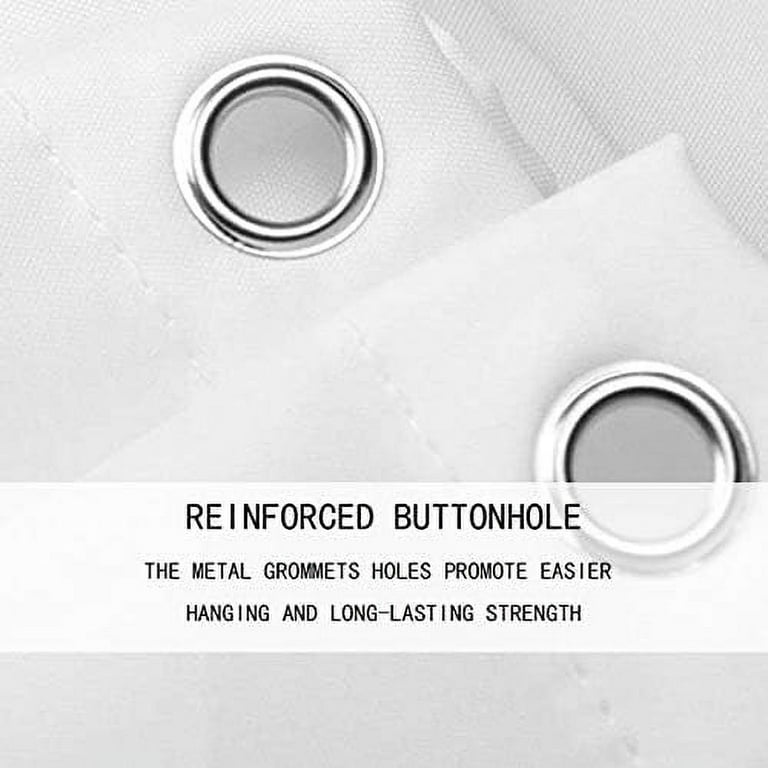The image is a close-up, zoomed-in photograph of a white, gauzy fabric material, likely a shower curtain or similar type of curtain, featuring two prominent metallic grommets. These grommets are cylindrical in shape, chrome in color, and are securely stamped into the fabric, providing reinforced buttonholes that promote easier hanging and long-lasting strength. The material around the grommets appears to be a white mesh-like texture. A white transparent banner with black capital letters overlays the center of the image, reading: "REINFORCED BUTTONHOLE. The metal grommets promote easier hanging and long-lasting strength." The fabric beneath the grommets has a seam and is angled towards the upper right of the image, emphasizing the durability and functionality of the grommets for holding up the material.